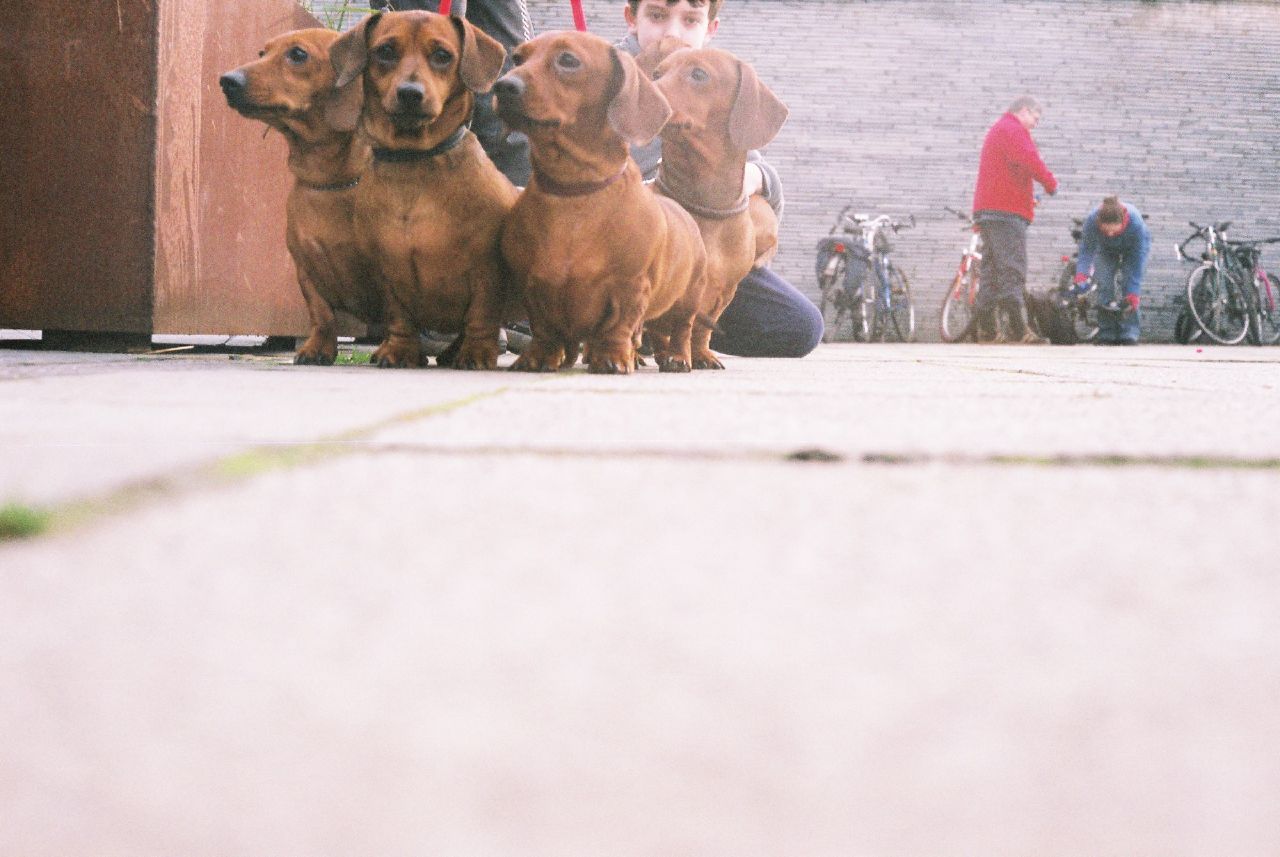This image captures four brown Dachshunds on a sidewalk, all leashed and held by a person just visible from the waist down. Each dog sports a different collar: a chain collar, a black collar, a red collar, and a round leather collar. The dogs are mostly facing off-camera, except one directly looking at the lens. Positioned closely behind them is a young boy with fair skin, who kneels, partially cut off at the top, and appears to be holding another Dachshund on his lap.

The background features a cycling scene with four or five parked bicycles. Two individuals, a man and a woman, interact closely by the bikes. The woman, identifiable by her hair in a bun and dressed in a blue shirt with red cuffs and jeans, is bending down. The man stands beside her, wearing a red long-sleeve jacket and black pants, possibly conversing with her. In this detailed composition, cracked cement tiles dominate the ground, contributing to the scene's urban atmosphere.